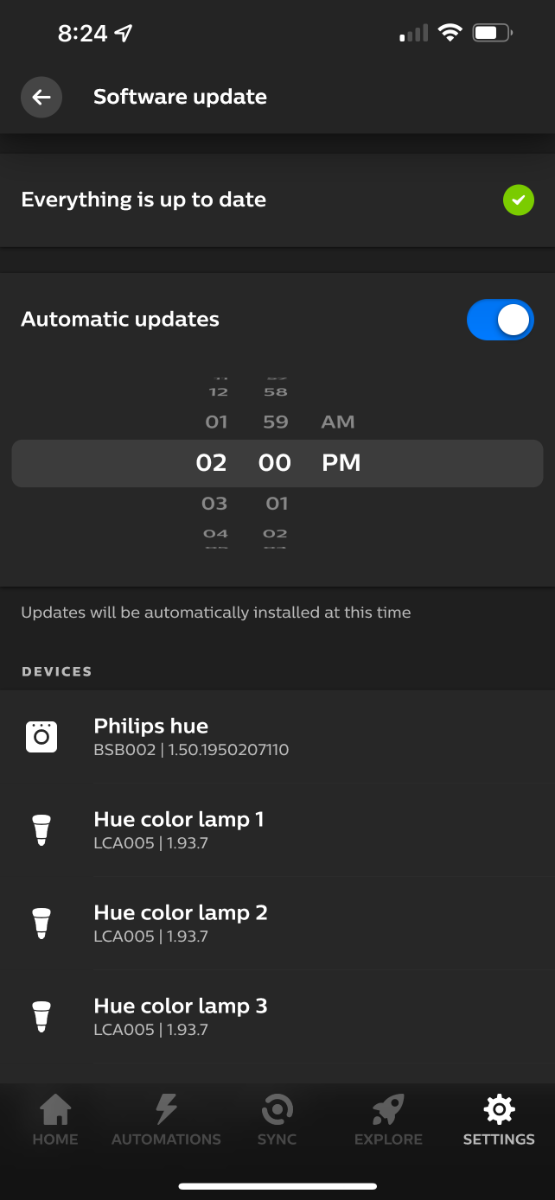The image is a screenshot from a phone displaying various settings. At the top left corner, the time reads "8:24". Directly below, a banner indicates "Software update" with a backwards-pointing arrow for navigation. The section underneath confirms that "Everything is up to date", accompanied by a green checkmark on the right.

In the subsequent section, "Automatic updates" are shown to be enabled, with the scheduled time set to 2 PM. A note clarifies that updates will be installed automatically at this time.

Further down, a list labeled "Devices" includes "Philips Hue" followed by "Hue Color Lamp 1", "Hue Color Lamp 2", and "Hue Color Lamp 3".

At the bottom of the screen, a row of buttons provides options: "Home", "Automations", "Sync", "Explore", and "Settings".

In the upper right corner, battery life is displayed slightly above half, full Wi-Fi signal strength is indicated, and the network signal strength shows one filled bar.